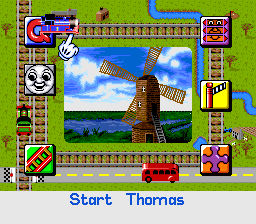This is a detailed screenshot from a vintage-style Thomas the Tank Engine video game. The central focus is a large, square-shaped section of railroad tracks set on a green grassy background. In the middle of the train tracks, there is a prominent windmill surrounded by grass, with a picturesque backdrop of a river, trees, and a blue sky dotted with clouds. Along the corners of the rectangular track area are various icons, including Thomas the Tank Engine and other colorful, cartoon-like characters with different facial expressions in shades of yellow, red, orange, purple, and blue. 

Adjacent to the tracks, at the bottom of the image, a road with yellow lines shows a red bus driving on it. Below this scene, the words "Start" and "Thomas" appear in blue, indicative of the game's interface. Additionally, there's a gray section featuring the text "Stark Thomas." The overall graphics exhibit a nostalgic 90s style, adding to the simple yet charming visual appeal of the game.